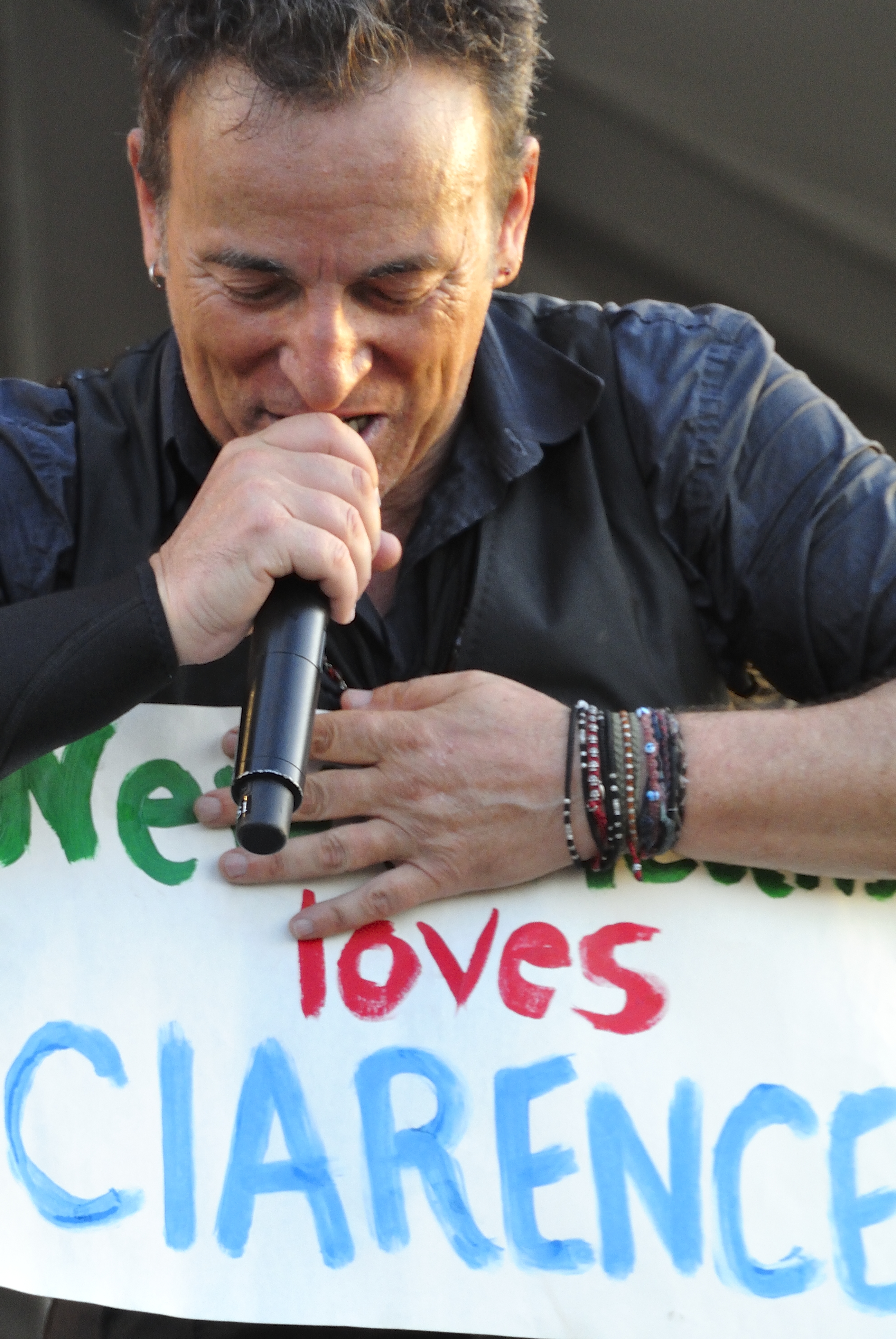In this image, Bruce Springsteen, the renowned rock musician, is seen holding a wireless microphone to his mouth. He is dressed in a black leather vest over a black shirt, his left arm bent at the elbow displaying numerous bracelets, likely between seven and nine. His right hand grips the microphone firmly. Springsteen's brown hair flows naturally as he looks down at a poster his left hand is holding. The poster, which features a white background, has large green letters "N-E" in the upper left corner, partially obscured by his arm. Below these letters, the word "loves" is painted in red, and underneath that, "Clarence" is boldly written in light blue letters, likely paying tribute to Clarence Clemens, a late member of his band. The setting features a gray curtain or wall material that serves as a subtle backdrop.